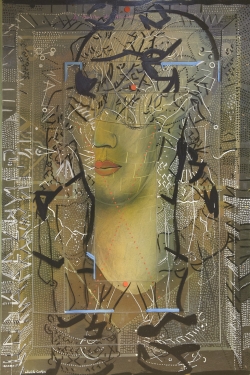This mixed media digital artwork presents an abstract rendition of a woman's bust, central to the composition. Dominating the canvas, the piece features a muted and moody palette primarily consisting of muted greens, browns, and darker black lines, with intricate white line designs that frame the subject like a border. Though abstract, the portrait conveys discernible features: a woman's neck, chin, coral red lips, and nose, but the eyes are obscured by repetitive line drawings, adding a sense of mystery. Her porcelain-like silhouette, aged to tan and dirty hues, is highlighted centrally, surrounded by a chaotic but harmonious assortment of lines and figures that mingle with textures of browns, blacks, and whites. The background predominantly brown, and interspersed details create a multi-layered and enigmatic ambiance. The composition suggests a figure emerging from, yet simultaneously dissolving into, abstract forms and scribbles that evoke hair cascading down, establishing a vivid but elusive representation of feminine identity and emotion.